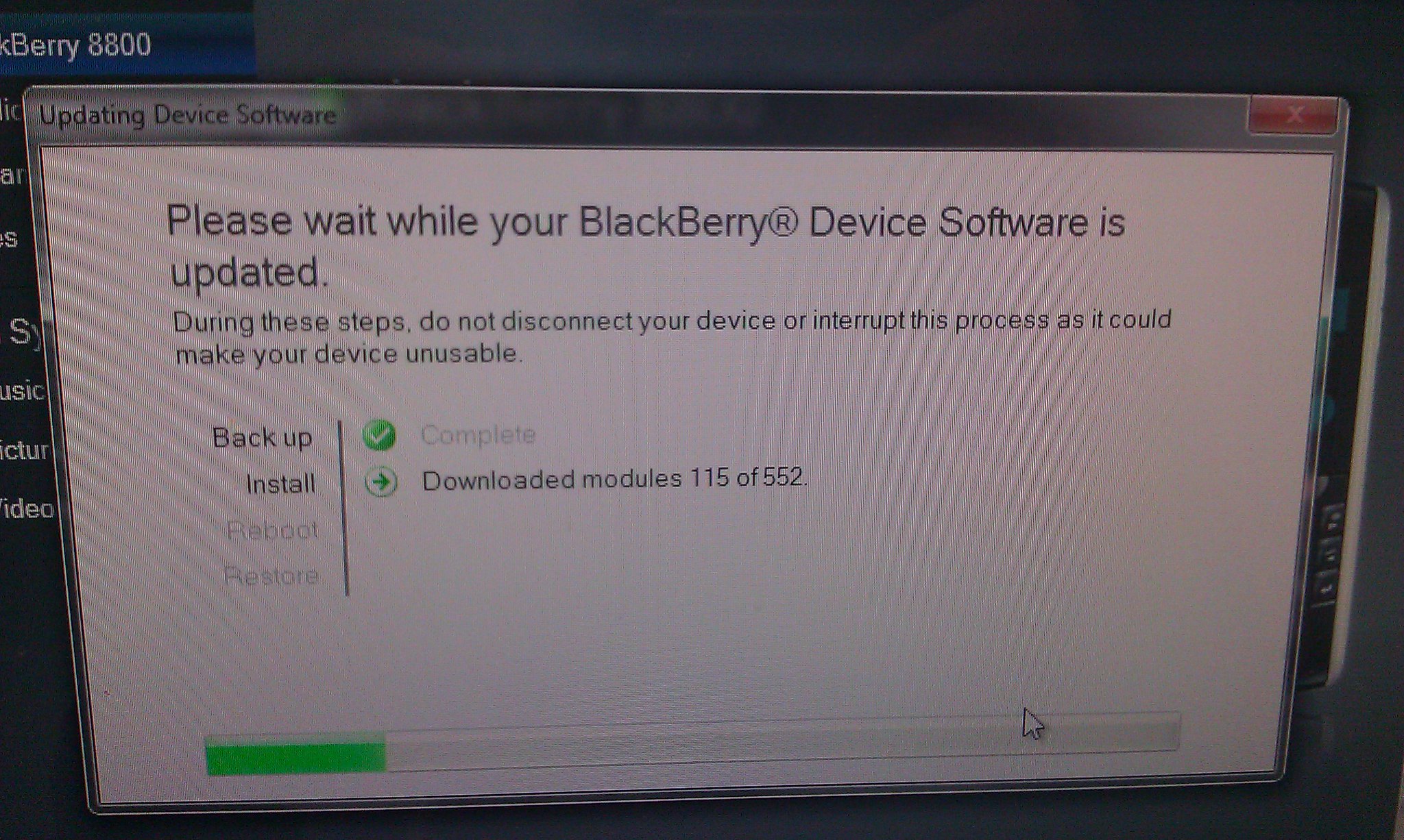This image is a photograph of a computer or laptop screen displaying a pop-up window for updating BlackBerry device software. The main screen behind the pop-up is slightly blurred. The pop-up window has a gray border and a white background, with the title "Updating Device Software" at the top left corner. In the top right corner of the window, there is a red X symbol.

Prominently displayed in the pop-up is the text: "Please wait while your BlackBerry device software is updated. During these steps, do not disconnect your device or interrupt this process as it could make your device unusable." 

On the left side of the window, there appears to be a column listing various stages of the update process. The stages mentioned include Backup (which is complete), Install (indicating downloaded modules 115 of 552, showing ongoing progress), with subsequent steps labeled as Reboot and Restore. At the bottom of the window, there is a green progress bar, which is approximately 20% filled, indicating that the installation is in progress. Additionally, a mouse pointer is visible near the progress bar.